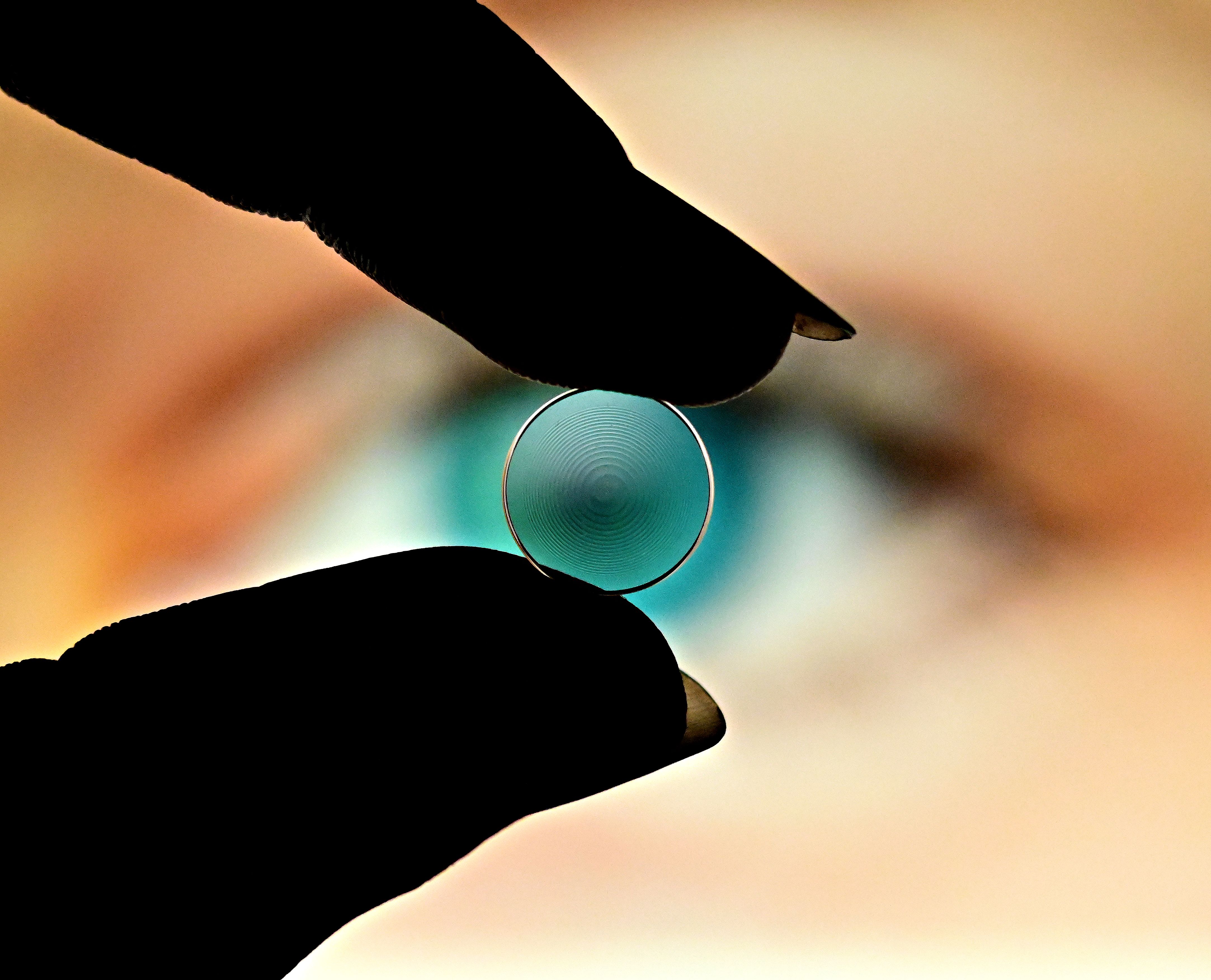In this highly detailed photograph, the focal point is a pair of fingers—thumb and index—holding a tiny, clear contact lens. The fingers, with long unpainted nails, are cast in deep shadow, appearing almost black, and are positioned prominently in the foreground. The lens, having an edge that almost seems gold in certain light, is perfectly centered, creating an illusion that aligns it precisely with the eye in the background. This eye, belonging to a fair-skinned individual, is a vivid, bright blue, almost turquoise, and despite being out of focus, adds depth to the image. The alignment suggests that the lens is about to be inserted into the eye, enhancing the composition's intricate detail and dramatic juxtaposition of light and shadow.